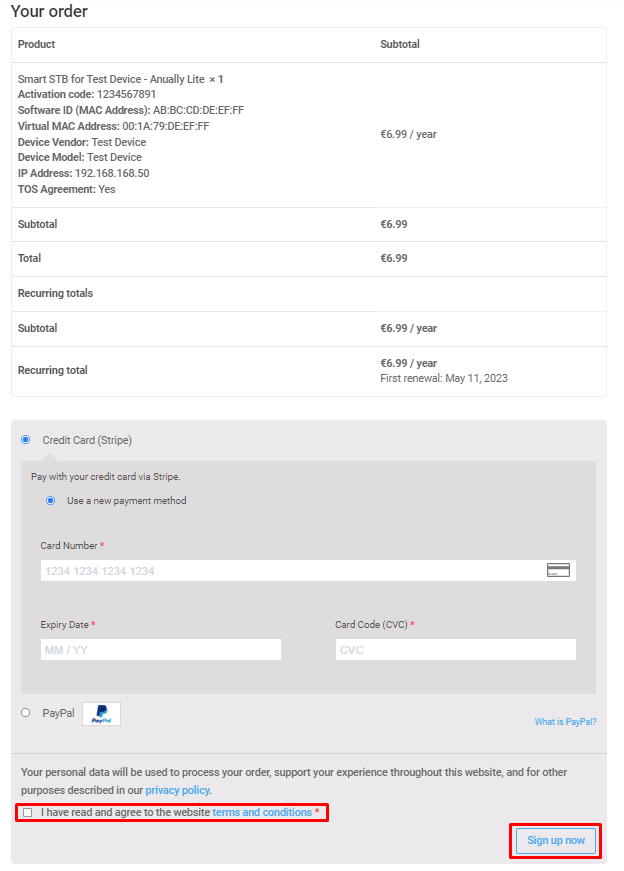This image is a clean screenshot set against a solid white background. In the upper left corner, there's the heading "Your Order." Beneath this, there's a light green banner followed by a light gray banner displaying "Product" and "Subtotal."

The main content details a subscription for "Smart STB for Test Device Annually," with a single activation code: "1234567891." Additional information includes the Software ID and the MAC address, with the following details:
- **MAC Address:** AABBCCDDEEFF
- **Virtual MAC Address:** 001A79DEEFF

Further down, it indicates the device vendor as "Test Device," priced at $6.99 per year. A faint gray horizontal line separates this section from the totals area.

The pricing summary lists:
- **Subtotal:** $6.99
- **Total:** $6.99
- **Recurring Total:** $6.99 per year